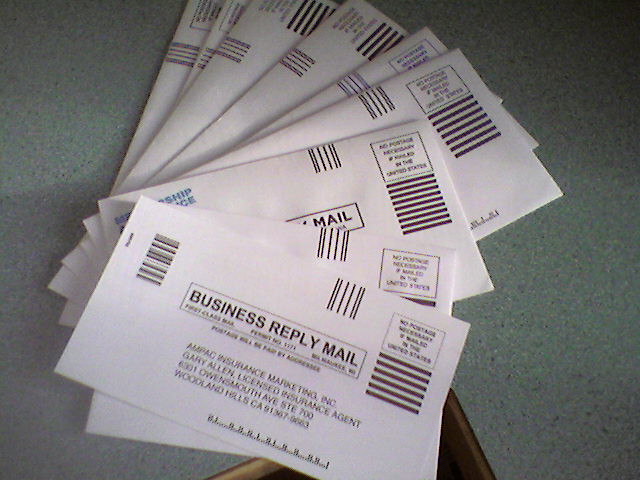This photograph captures a neatly fanned-out stack of business reply mail, all featuring identical white envelopes with a distinct square in the top right corner marked "No Postage Necessary". Each envelope prominently displays "Business Reply Mail, First Class" and is addressed to Ampag Insurance Marketing Incorporated, Gary Allen Licensed Insurance Agent, located at 6301 Owens Mouth Avenue, STE 700, Woodland Hills, California, 91367-9663. The envelopes, laid out in a fan-like arrangement on a teal or light green tabletop, make the repetition of the design and address particularly striking. The scene is uniformly lit, emphasizing the consistent patterns of bars under the postage square and the uniformity of the business reply mail envelopes.